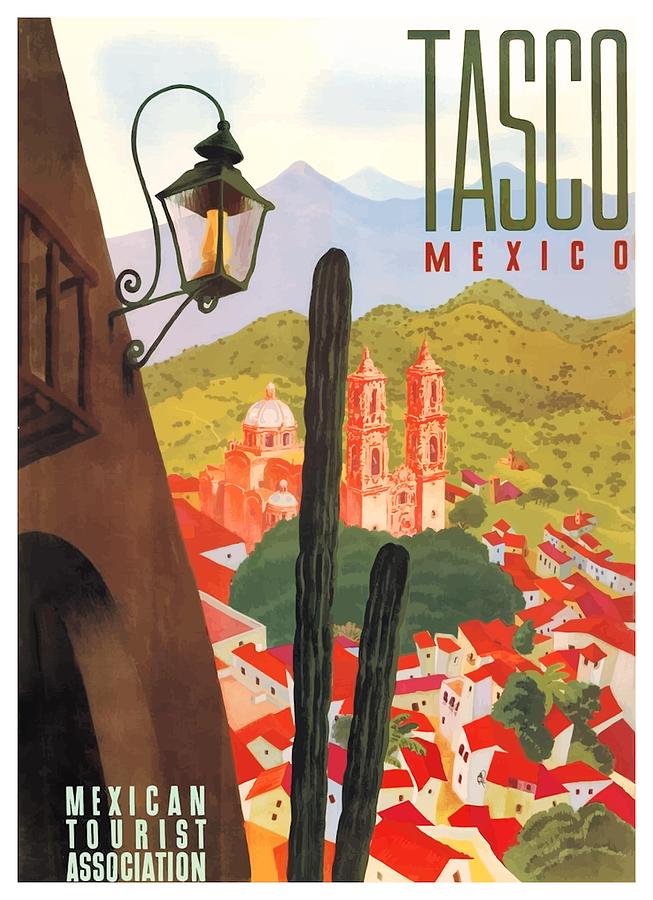This vintage-style poster, advertising for the city of Taxco, Mexico, carries a sense of nostalgia with its muted yet bright colors. Dominating the top, "Taxco" is written in a green, sage-like hue, with "Mexico" in bold red letters beneath it. The central image is an artistic interpretation, possibly computer-generated, showing a high vantage view of Taxco. 

A large, tall cactus stands prominently in the foreground beside an adobe building adorned with an ornate, black wrought iron light fixture that emits a soft yellow glow. This building’s brown exterior and stairs add to the rustic charm. The scenic vista reveals white buildings with traditional red roofs nestled among sporadic trees, presenting a picturesque townscape. A grand cathedral is a focal point within the city.

The background features layers of mountains: a near range colored in yellow with tree coverage and a further range in blue, accentuating the depth of the landscape. The sky above is primarily white, punctuated by a few circles of blue, hinting at a clear day with scattered clouds. This evocative scene is bordered at the bottom by the inscription "Mexican Tourist Association," indicating the poster’s purpose of promoting tourism.